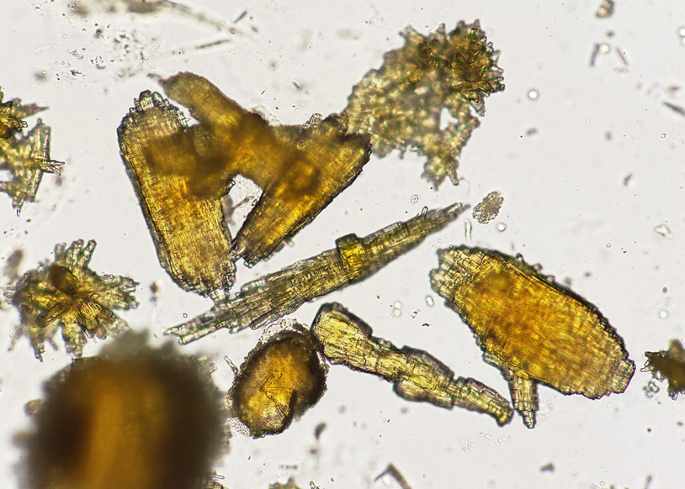This image displays a magnified view of amber-colored crystalline structures on an off-white background, reminiscent of a scene under a microscope. The particles vary widely in shape and size, ranging from jagged crystals to shard-like fragments, some resembling pieces of glass or cracked tree bark. The colors span from a dark golden brown to a lighter butterscotch or honey shade, with some elements appearing more translucent, allowing for layers to be visible. Many of these structures possess sharp, irregular edges, and their arrangement appears random, scattered across the field of view. There are also smaller particles and bubbles interspersed among the crystals, adding to the complexity of the scene. A noteworthy detail is that parts of the image, particularly in the bottom left, seem out of focus, possibly due to moisture or an incorrectly adjusted lens. Overall, the well-lit composition highlights the intricate textures and the crystal-like appearance of these curious, amber-toned particles.